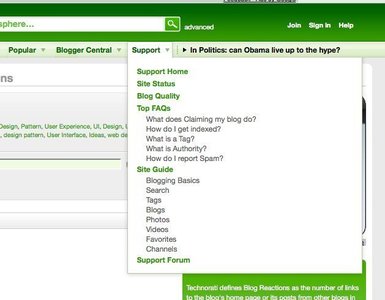The image displays the right half of a web page with the left side cut off. At the top, there is a bright green ribbon spanning across the page. Partial visibility of a search box can be seen towards the left side of this section. Adjacent to the right of the search box, 'advanced' is written in lowercase white letters, followed by options for 'join,' 'sign in,' and 'help' aligned to the far right.

Beneath this top bar is a thin, light gray banner highlighting different navigation options. The visible options include 'popular,' 'blogger central,' and 'support,' with 'support' being selected. A dropdown menu appears under 'support,' listing several items in dark green text: 'support home,' 'site status,' 'blog quality,' and 'top FAQs.'

Following these items in gray text are further options: 'what does claiming my blog do,' 'how do I get indexed,' 'what is a tag,' 'what is authority,' 'how do I report spam.' The green text item 'site guide' appears next, followed by more options in gray text: 'blogging basics,' 'search,' 'tags,' 'blogs,' 'photos,' 'videos,' 'favorites,' and 'channels.' The dropdown concludes with 'support forum' in green text at the bottom.